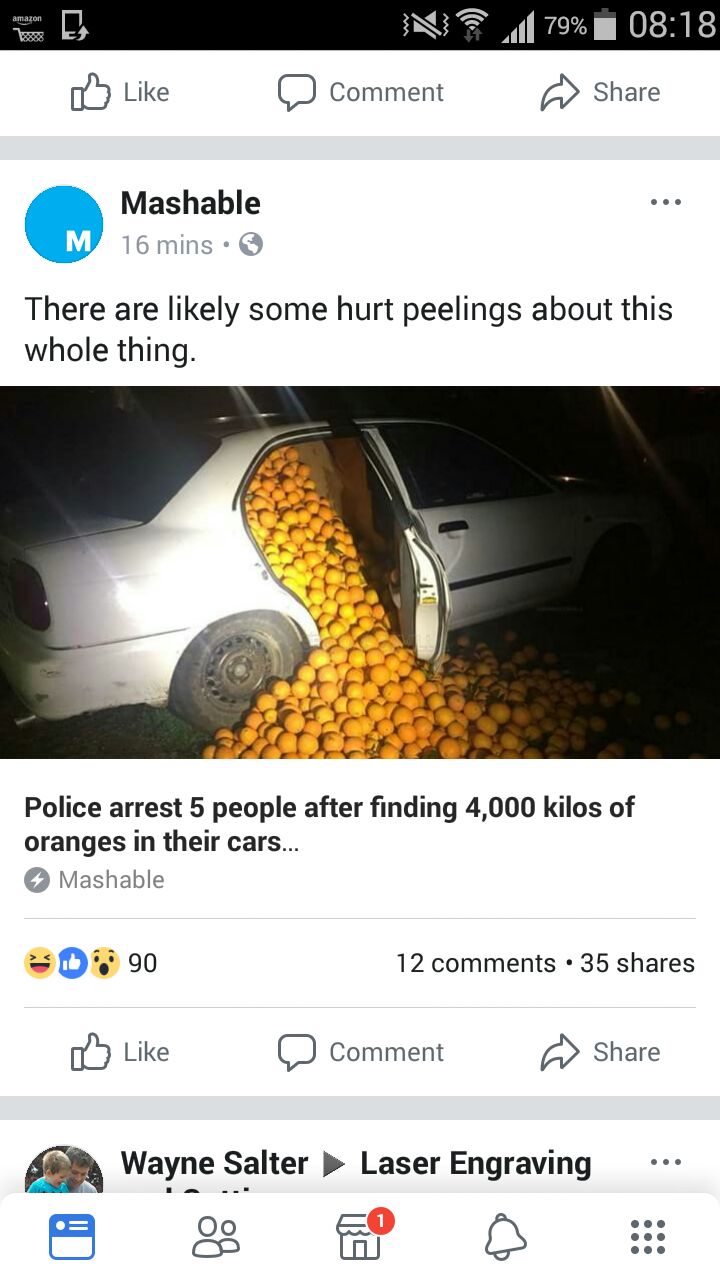The image is a screenshot of a mobile phone displaying a Facebook feed featuring a post from Mashable. The phone shows the time as 8:18 and battery life at 79%. The highlighted Mashable post, identified by its blue circle logo with a white 'M', was shared 16 minutes ago. The meme reads, "There are likely some hurt peelings about this whole thing," and features a picture of a white 90s sedan with its back door open, spilling numerous oranges onto the ground at nighttime. The post's headline states, "Police arrest five people after finding 4,000 kilos of oranges in their cars." Below the image, there are reactions from users, including laughter, shock, and thumbs-up emojis, totaling 90 reactions along with 12 comments and 35 shares. At the bottom of the screenshot, unrelated to the meme, there is a partial view of another post mentioning "Wayne Salter, laser engraving." The Facebook interface is in daylight mode with a white background, and the notification bar at the bottom shows a home icon with a red notification indicator.